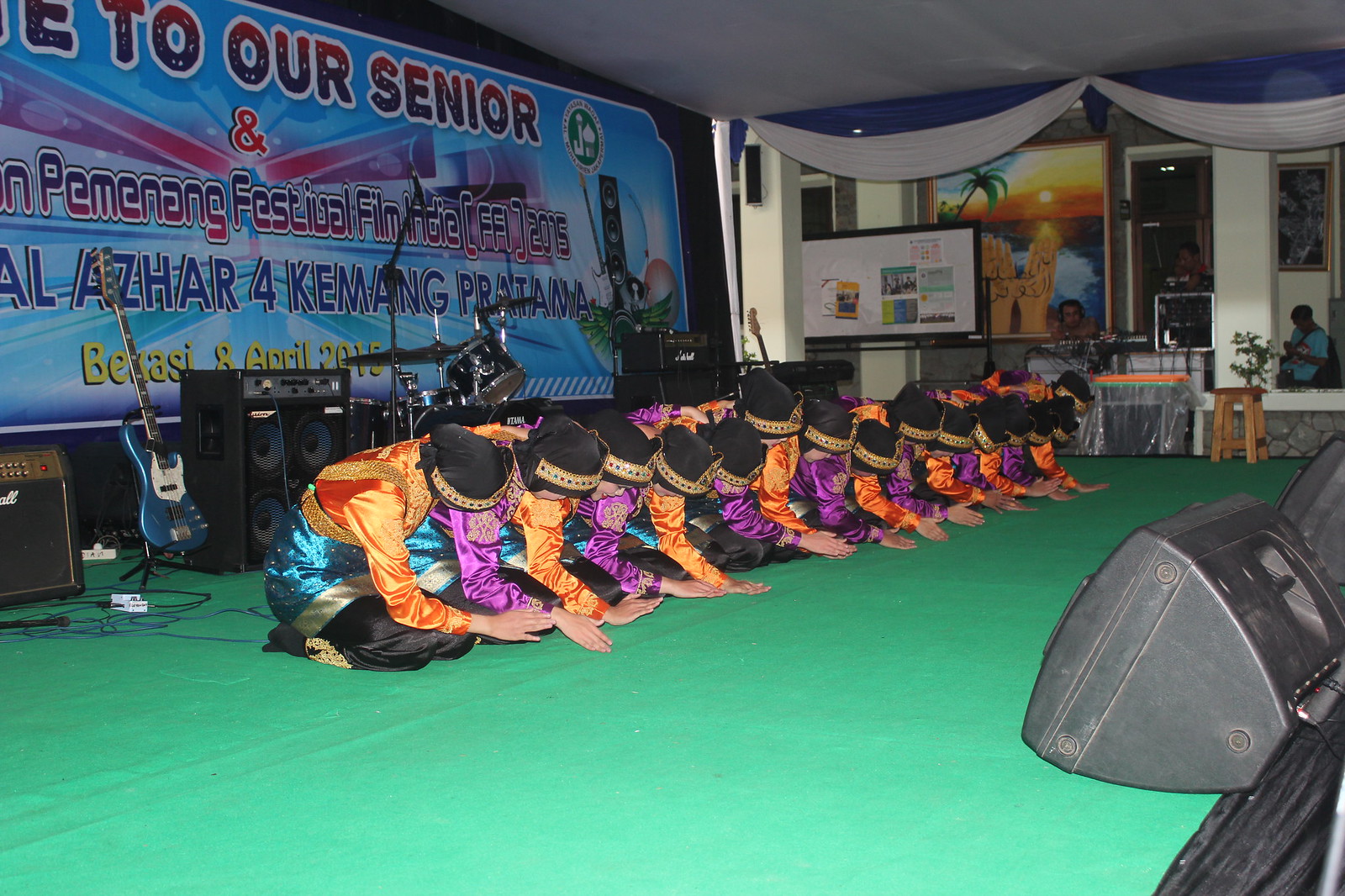This photograph depicts a group of approximately 14 to 15 individuals, possibly monks or holy figures, dressed in a variety of colorful robes that include light mint green, several shades of blue, red, black, white, yellow, orange, and purple. They are kneeling on a raised stage with green flooring, their hands extended forward in a pose that suggests prayer or a ritual. Behind them, there's a partially visible sign with a blue background featuring text in both English and another language, which includes phrases like "to our senior" and "Penang Festival Film Indie FF 2015 Azar for can make Prathama." The backdrop of the stage is adorned with musical instruments, such as a blue and white guitar and drums, as well as potential stage lighting or speakers on the right side. The entire scene is framed by a picturesque sunset with a palm tree, replete with hues of green, orange, yellow, and tan, underscoring the serene yet vibrant atmosphere of the event.